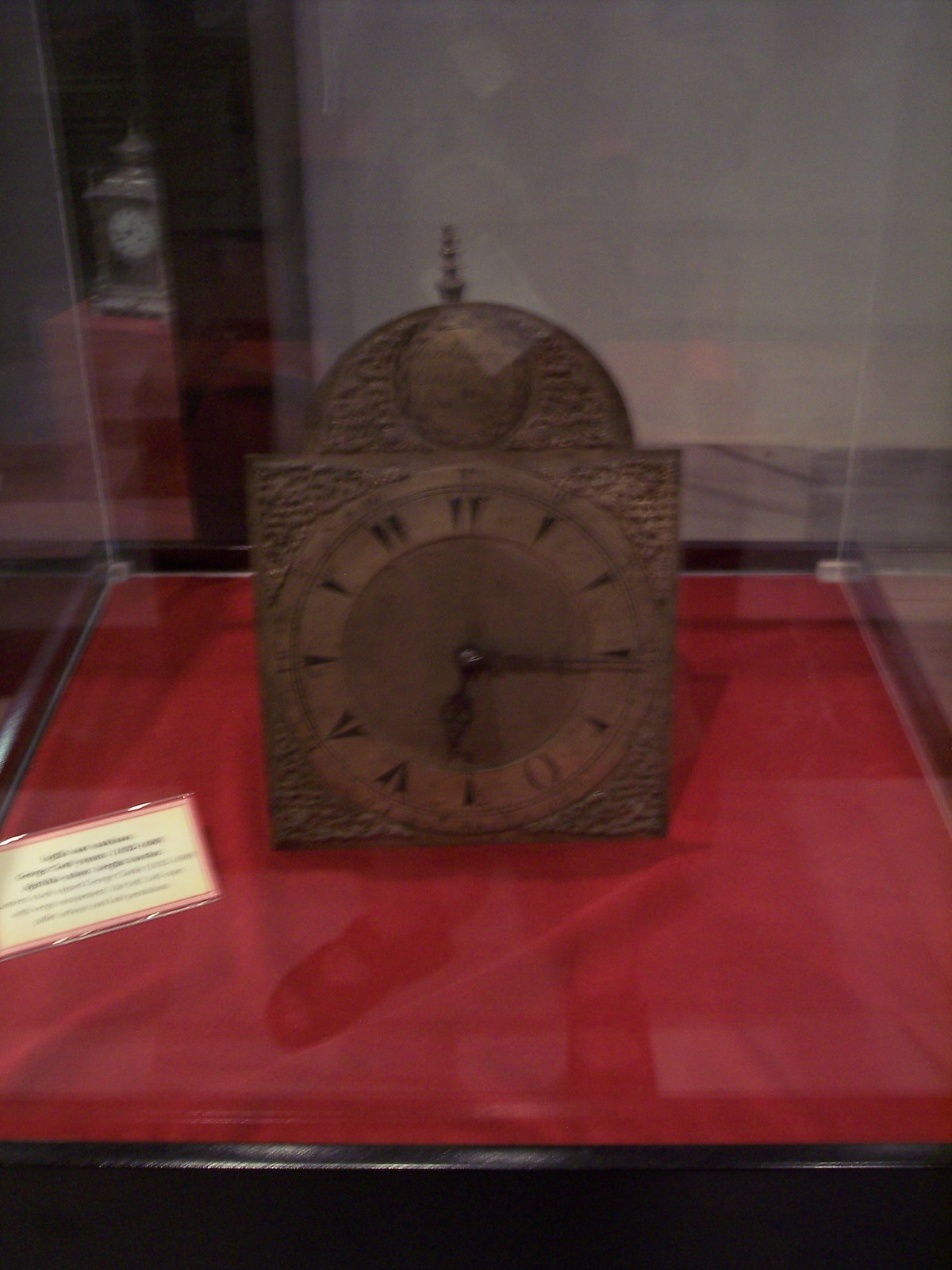The image depicts a museum exhibit featuring an antique clock displayed inside a glass showcase cabinet. The clock rests on a red cushion positioned on a black base. The clock itself is predominantly brown with some darker patches and appears to be made of a metal like bronze or copper, though its exact material is indeterminate. The design of the clock includes a square base with a circular face, and atop it, a dome featuring a circular element in its center. This clock is adorned with symbols instead of conventional numerals, with dark metal hands indicating time.

Accompanying the clock is a small, blurred informational card or label, likely containing details about the artifact, though the text is unreadable. The lighting and reflections on the glass case reveal the shoes of the person who took the photograph, hinting at a summer visit, as they appear to be sandals. 

In the left background, another clock is visible, also encased in glass and sitting on a red cushion. This additional clock has a lighter gray tone with some darker patches, suggesting it too might be of significant historical value and crafted from different materials. Both exhibits together imply this could be part of a specialized clock museum or a section dedicated to timepieces within a larger museum.